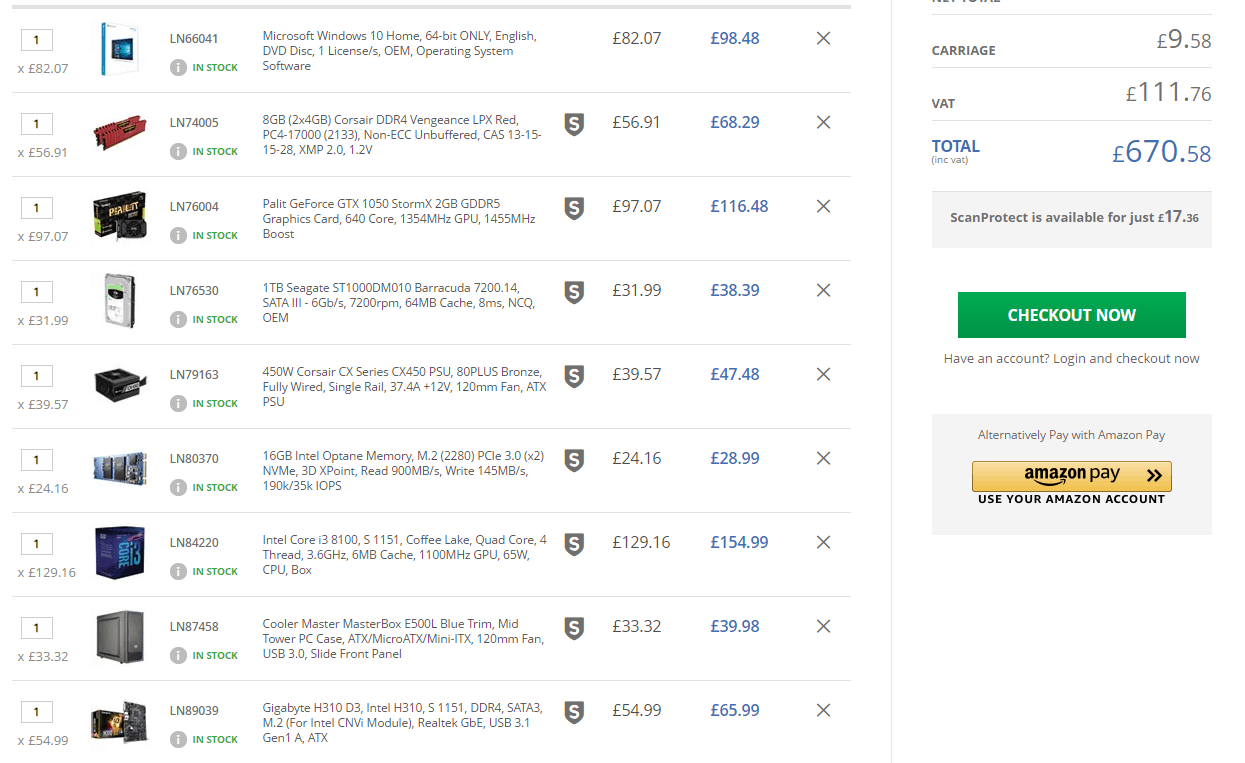The image displays a detailed webpage where various computer components are available for purchase. There are nine different parts listed, each accompanied by an image on the left:

1. At the top, a **Microsoft Windows 10 64-bit DVD** writer, priced at £98, offering an essential operating system for PC users.
2. Below that, a **Corsair Vengeance DDR4 RAM module** at £68—this appears to be a memory module rather than a video card.
3. Next, a **Palic GeForce GTX video card** is listed for £116, providing robust graphics capabilities.
4. Moving down, a **1TB Seagate Barracuda HDD** with a 64MB cache is available for £38, offering ample storage.
5. Below that, a **450W Corsair Series Bronze Fully Wired Single Rail Power Supply** is priced at £47.48, ensuring power efficiency and stability.
6. The next item is a **16GB Intel Optane Memory Module**, priced at £28.99, which enhances data access speeds.
7. Following, an **Intel Core i5 Coffee Lake Quad Core Processor** with 4 threads and 6MB cache, priced at £154.99, is shown for efficient processing.
8. Below that, a **Cooler Master MasterBox Blue Trim Tower PC Case** is available for $39, offering a stylish and practical housing for the components.
9. Finally, a **Gigabyte Intel H310 Motherboard**, supporting DDR4 memory, is listed at £65.99, providing a solid foundation for system builds.

Each component is clearly depicted and well-detailed, providing potential buyers with all the necessary information to make informed purchasing decisions.